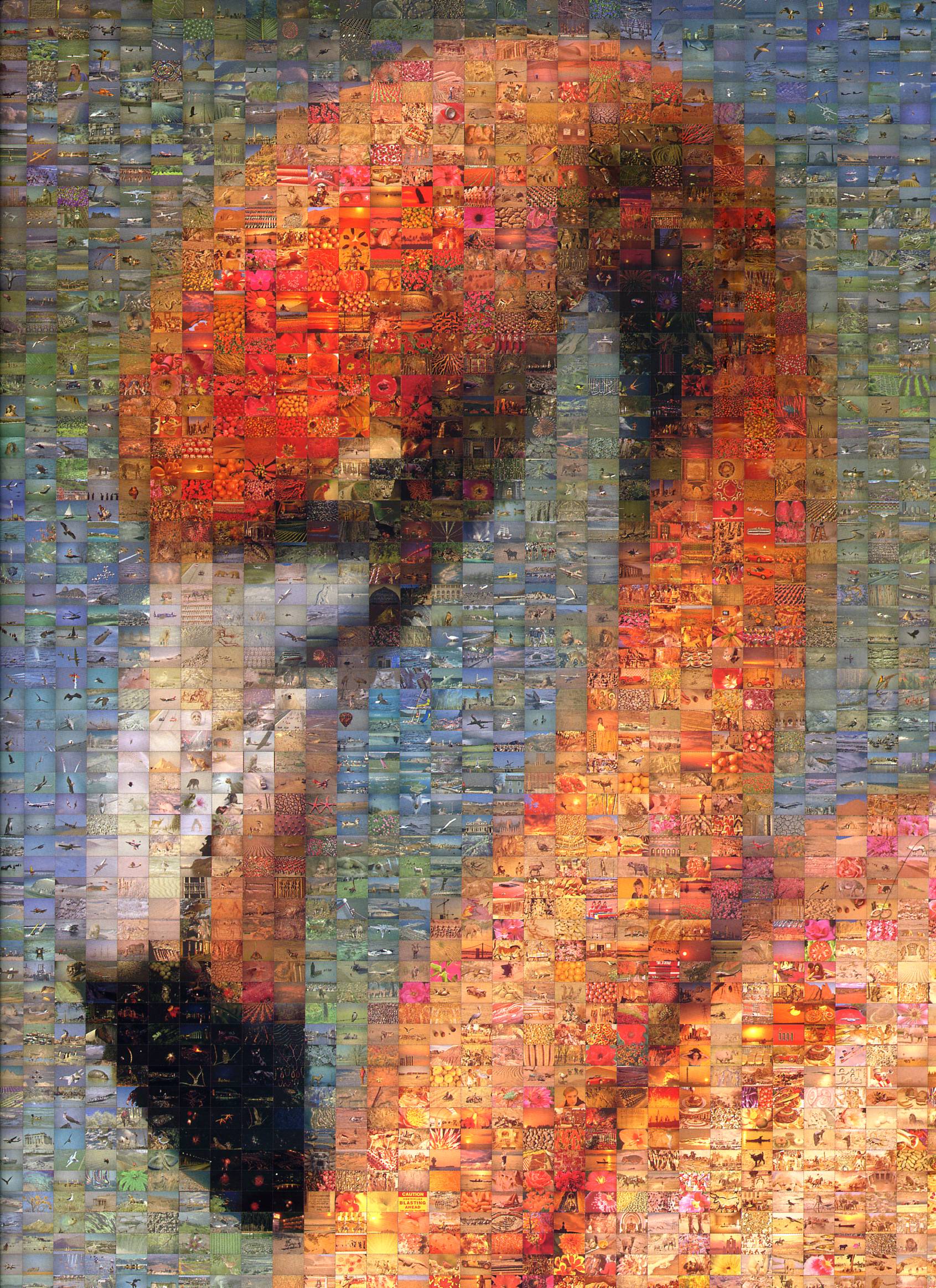This artwork is a highly detailed composite image of a flamingo's head and neck, created from hundreds of tiny individual pictures. Each small rectangle, resembling mini screens, contributes to the overall depiction, forming a mosaic-like grid that intricately blends together to form the flamingo. The bird's distinct features—a dark pink head, sweetheart-shaped arched neck, and a beak that's light pink with a black tip—are clearly visible. The flamingo appears against a green and blue background composed of similarly toned images, enhancing the textured and pixelated appearance of the entire artwork. When viewed up close, the image reveals a tapestry of diverse subjects, including flowers, sunsets, various nature scenes, beaches, boats, and even whales, strategically chosen to match the color spectrum of the flamingo and its background. The eyes of the flamingo are yellow, adding a striking contrast to the composite image. The overall picture is slightly blurry, further contributing to the illusion of a single cohesive portrait when seen from a distance, yet unveiling a multitude of smaller, vibrant worlds upon closer inspection.